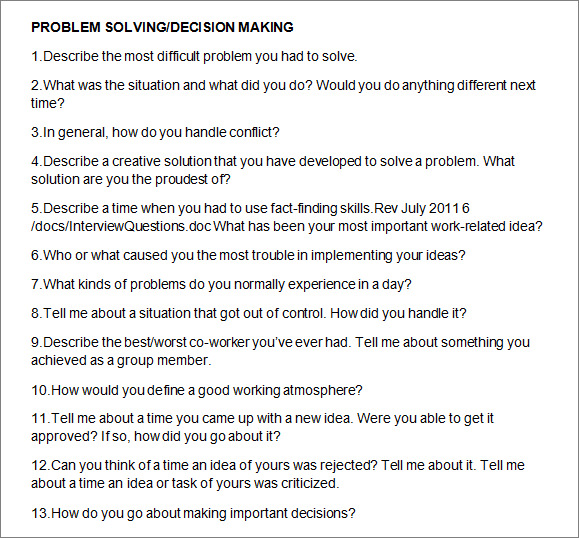This image is a screenshot taken from what appears to be a guide on problem-solving and decision-making, presented on a clean, white background with black text. The title of the webpage, located at the top left corner, is "Problem Solving / Decision Making."

The content is organized into a list of numbered steps, ranging from 1 to 13, designed to lead readers through various aspects of tackling complex problems and making important decisions. Here are some key points from the guide:

1. "Describe the most difficult problem you have had to solve."
2. "What is the situation and what did you do? Would you do anything different next time?"
3. "In general, how do you handle conflict?"
4. "Describe a creative solution that you have developed to solve a problem. What solution are you the proudest of?"

Further down the list:

7. "What kinds of problems do you normally experience in a day?"
8. "Tell me about a situation that got out of control. How did you handle it?"
13. "How do you go about making important decisions?"

This guide is designed to teach individuals how to effectively approach problem-solving and decision-making. It provides a structured method to reflect on personal experiences, handle conflicts, develop creative solutions, and manage daily challenges, ultimately aiding in the enhancement of decision-making skills.